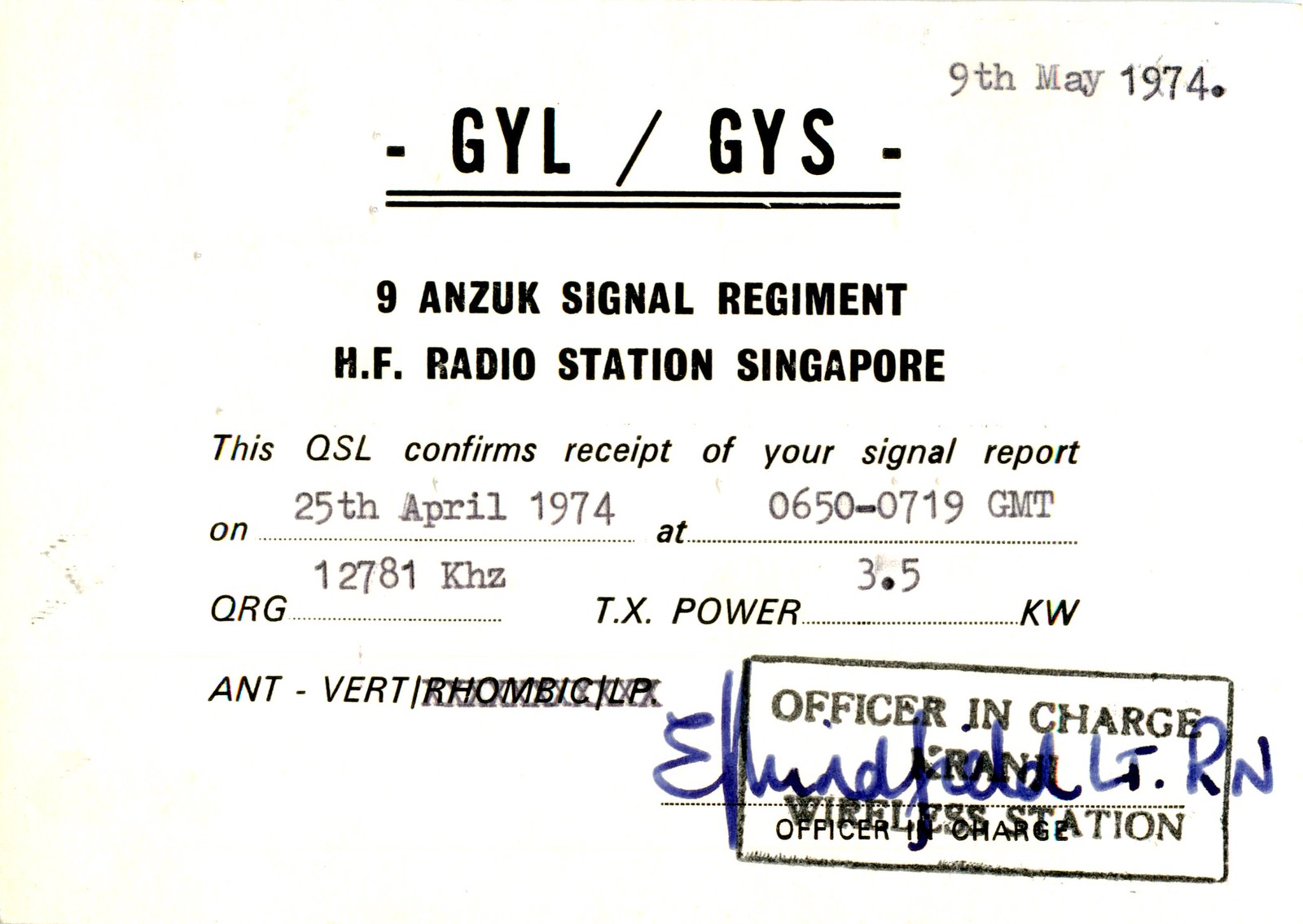This square image features an all-white background filled with letters, numbers, and dates, resembling a certificate or receipt. In the upper right, the date "9th May 1974." stands out. Centered at the top, there is a header reading "GYL/GYS" followed by "9 ANZUK Signal Regiment." Directly below, it reads "H.F. Radio Station Singapore." The middle section of the image contains the text, "This QSL confirms receipt of your signal report on 25th April 1974 at 0650-0719 GMT, QRG 12781 KHz, T.X. power 3.5 KW, ANT-VERT." Toward the bottom right, a stamp reads "Officer in Charge," next to which a blue signature indicates "Wireless Station." This document appears to certify the reception of a signal report from a historical radio communication event.